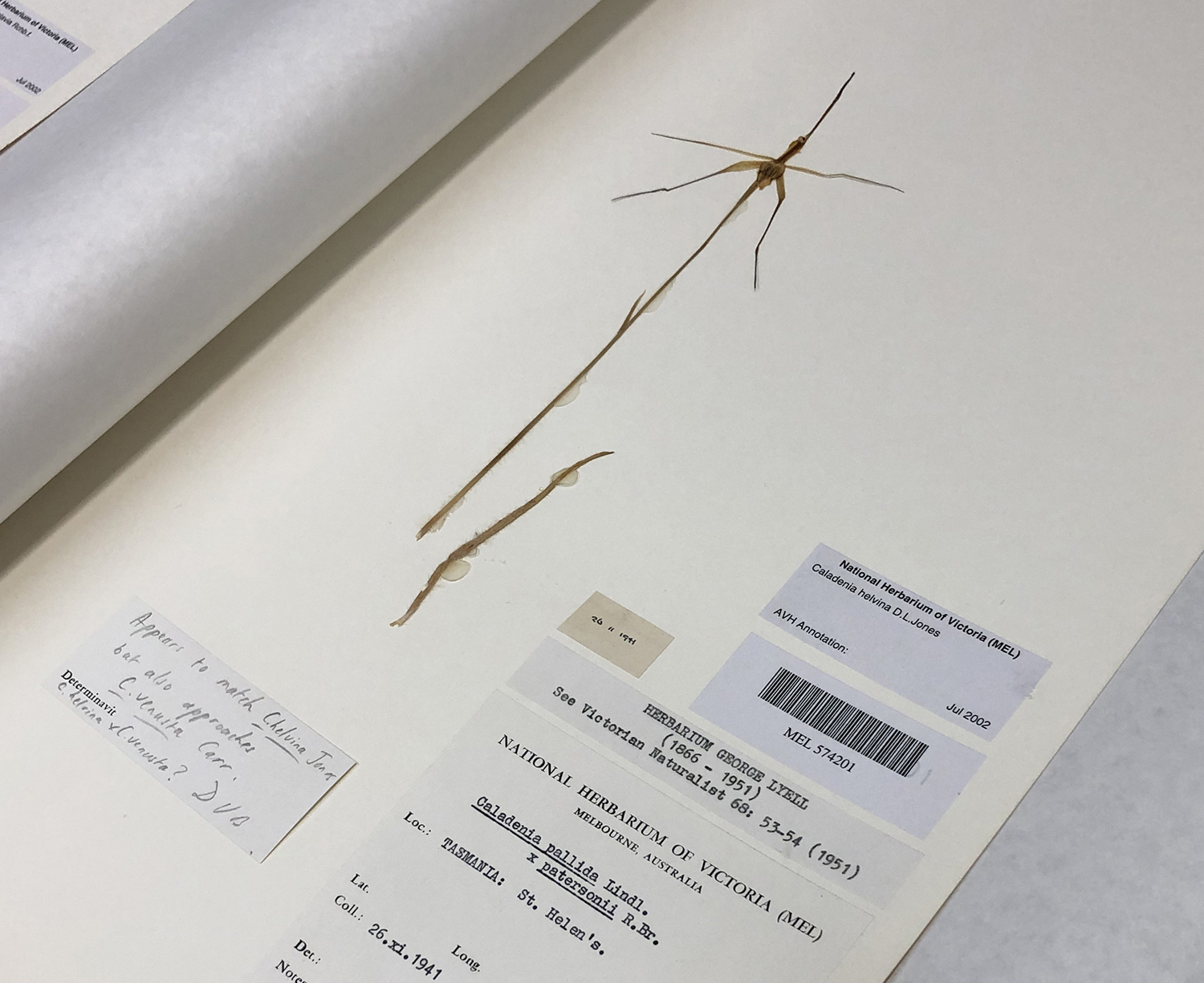A detailed specimen of a plant arranged on a large piece of cardstock is showcased in the center of this image. The plant features a brown long stem that branches out in a cross-like pattern, with additional slender stems resembling cricket legs, meticulously glued onto the card. A smaller, unattached stem is also present. The cardstock is adorned with various labels and stamps that provide detailed information. One label reads, "National Herbarium of Victoria M.E.L., Caledonia Hevna D.L. Jones, AVH Annotation, July 2002." Below this, there is a barcode labeled MEL 574201. Another small brown piece of paper reveals that the specimen dates back to October 20, 1941, from the Herbarium George Lyell, who lived from 1866 to 1951 and was a renowned Victorian naturalist. Additionally, a post-it note indicates a potential identification, mentioning the plant matches "Chalvena Jones" but also closely resembles "C. Venita Carr." This carefully preserved and documented specimen underscores its archival and botanical significance.